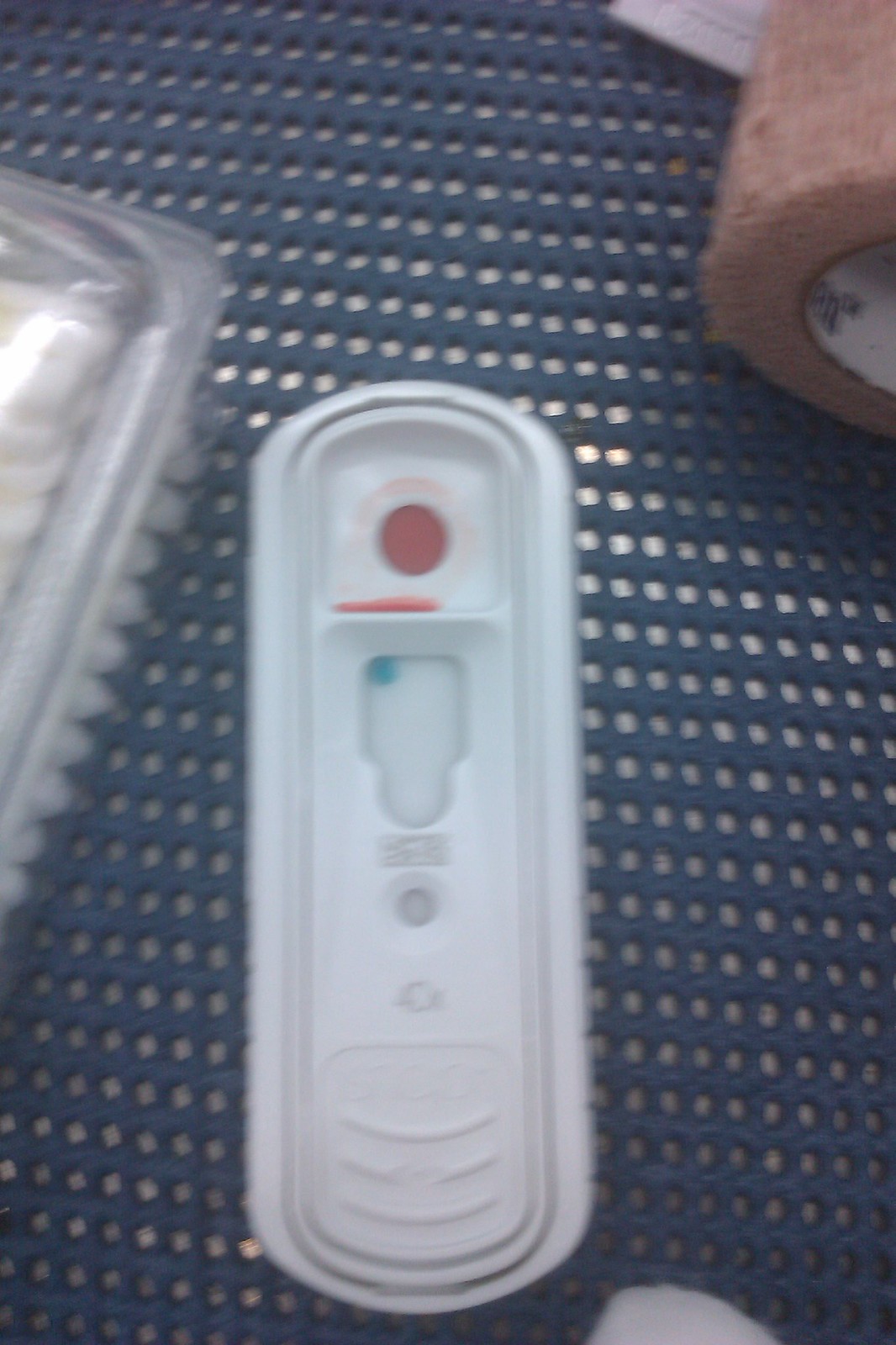The image features a somewhat blurry scene with a blue mesh background characterized by small, uniform holes. Central to the composition is a white, rectangular object with rounded ends. This object has a circular red mark near its top, with three lines etched at its base, and a small green dot located just beneath the red circle. In the top right corner, a tan-colored roll of bandage is partially visible, accompanied by a piece of paper that is cut off at the edge of the frame. On the left side of the image, there's a clear package containing an item with white bristles; this item is of a comparable size to the white object in the center. The exact nature of these objects is unclear, suggesting they may be some form of equipment.